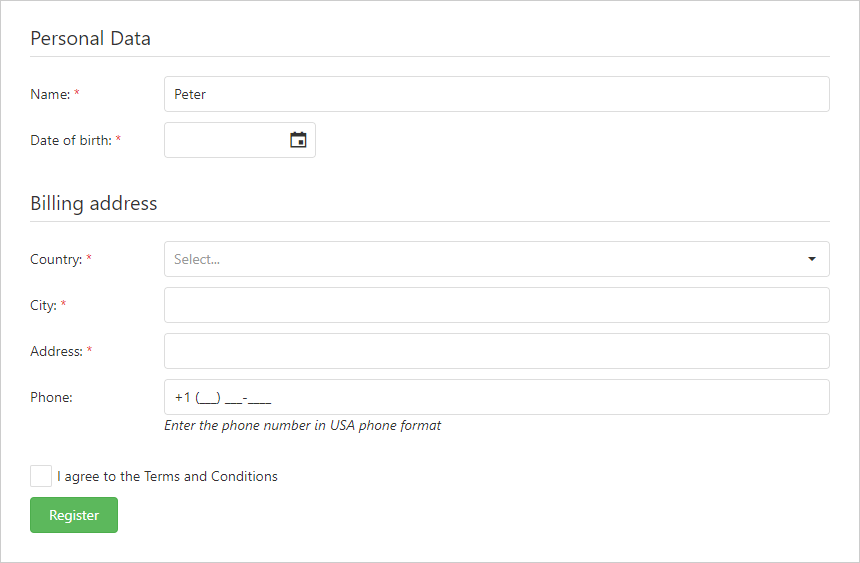In this image, we observe a detailed data entry form designated for personal information. At the top, a header in black and white reads "Personal Data." Directly below this header, there is a section for "Name" with a corresponding input box that has "Peter" already entered. The following section pertains to "Date of Birth," accompanied by an input box with a calendar icon, likely allowing the user to select a date via a calendar interface.

Continuing downwards, the form addresses "Billing Address." The first entry in this section is labeled "Country," featuring a clickable drop-down menu for selection. Below this, there is a space labeled "City" with an input box intended for text entry. Further down, the form requests an "Address," once again with a text entry box for detailed information.

Subsequently, there is a field for "Phone" with an input box for a phone number entry. Notably, beneath this field, there is a guideline indicating to "enter the phone number in USA phone format." At the bottom of the form, a checkbox labeled "I agree to the terms and conditions" is present, signifying user consent. The form is concluded with a prominent green "Register" button, inviting users to submit their details.